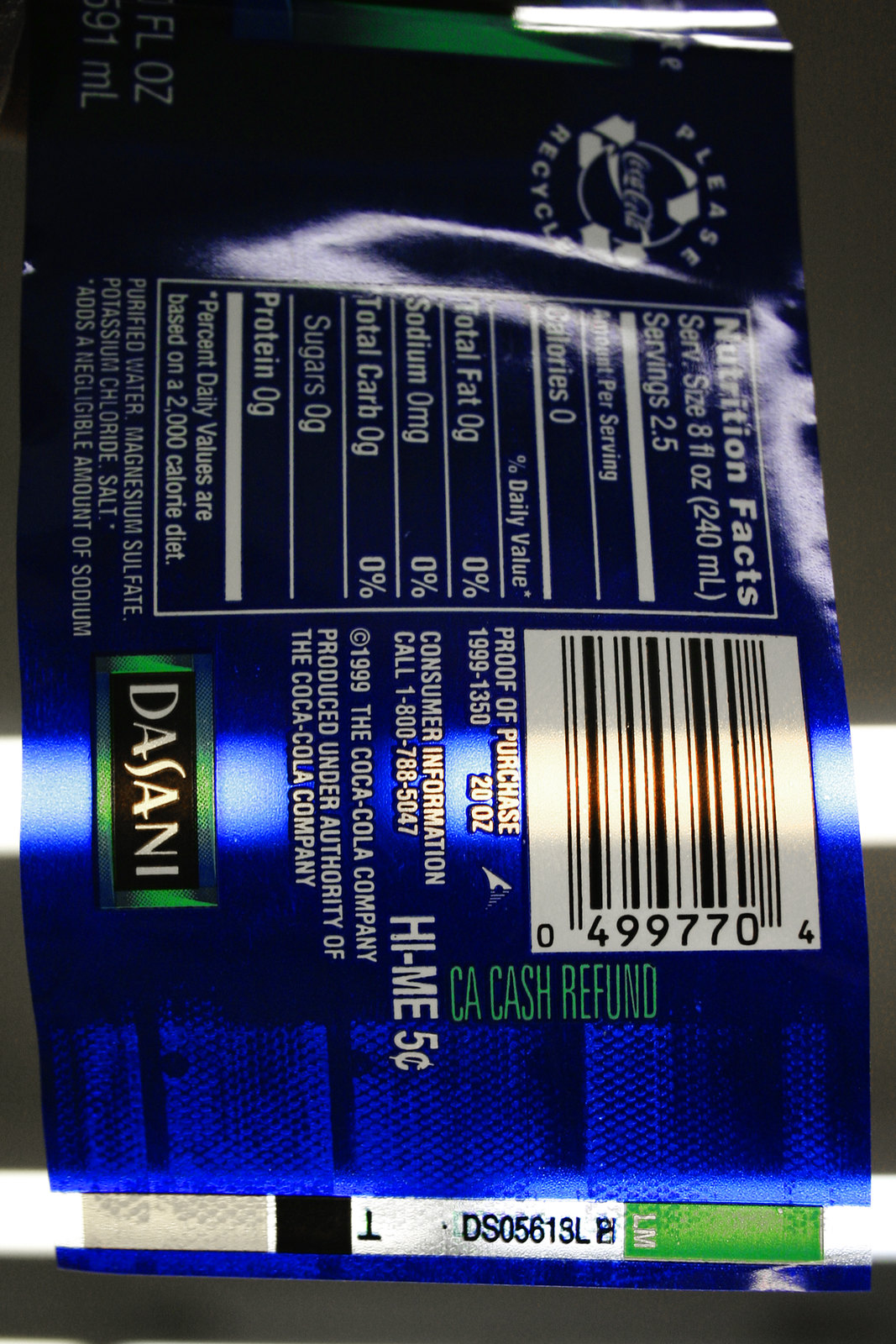The image features a laid-out, unwrapped Dasani water bottle label, showcasing its detailed design and nutritional information. The label, which is no longer wrapped around the bottle, is set against a backdrop with fluorescent lights cutting across near the bottom. Dominated by a light reflective blue color, the Dasani logo stands prominently on the left side. The nutrition facts box, also on the left, is oriented vertically and lists zero calories, total fat, sodium, total carbs, sugars, and protein, reflective of typical water nutritional content. Additional details include a green font barcode with a 'CA cash refund' notation and the 'Please Recycle' message intertwined with the Coca-Cola logo and recycling symbol. The year 1999 is marked, indicating the Coca-Cola company, and at the very bottom, there is a white horizontal strip bordered with green and black, containing miscellaneous information.